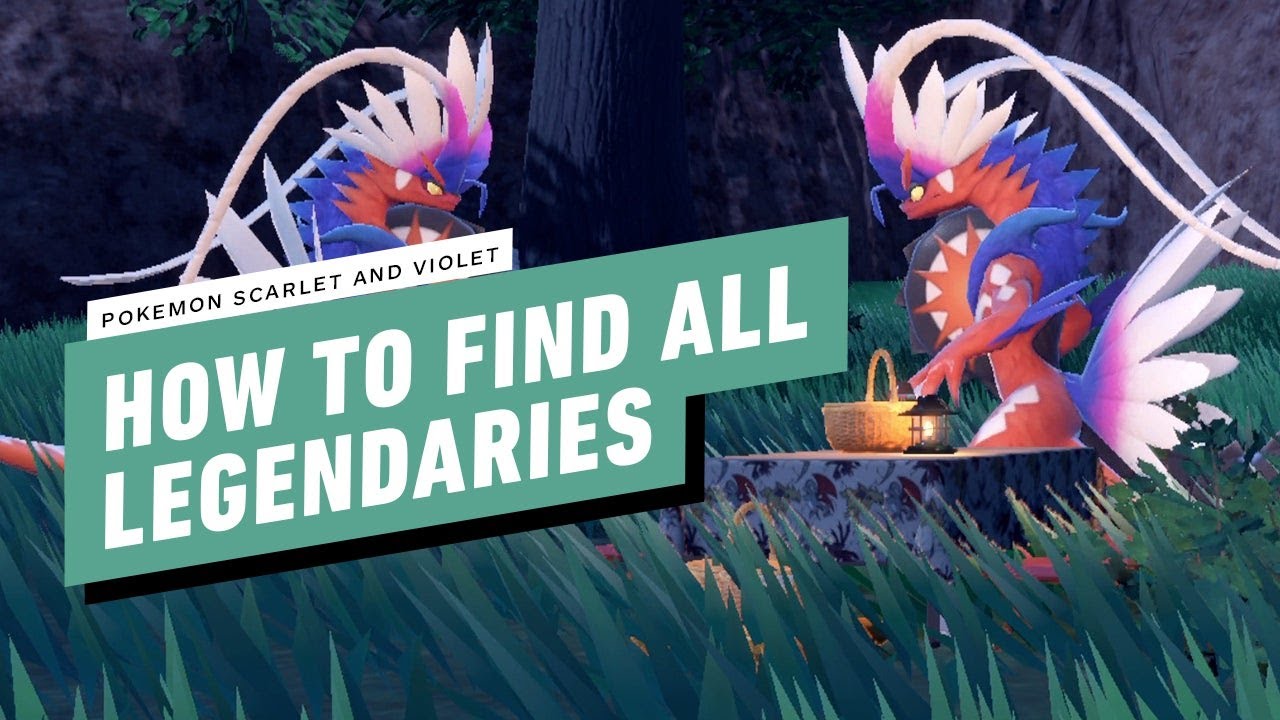The image is a poster with a green background and detailed illustrations. At the top, a green sign with white writing boldly states, "How to Find All Legendaries." Above this sign, another smaller white sign with black text reads, "Pokemon Scarlet and Violet." Below these signs, the poster appears to showcase a landscape with painted grass in two shades of green, evoking a forest-like setting. On the right side of the image, there is a prominent depiction of a Pokemon creature, characterized by its intricate features: it has a red and orange body with sharp, dinosaur-like spikes along its back, large white and red tentacles or feather-like extensions from its head, and a basket in front of it. The creature also sports an array of colorful feathers—blue, violet, and white—protruding from its tail area, with these vibrant hues blending into shades of pink and purple. Above the "Pokemon Scarlet and Violet" sign, a partial view of the same creature is visible, showing it from below the head area and upwards. Both figures seem to be gazing at each other. The background includes darker shades suggesting trees, enhancing the forest atmosphere but making the details less distinct. The overall text is primarily white, with "How to Find All Legendaries" in green and white, and "Pokemon Scarlet and Violet" in black and white.